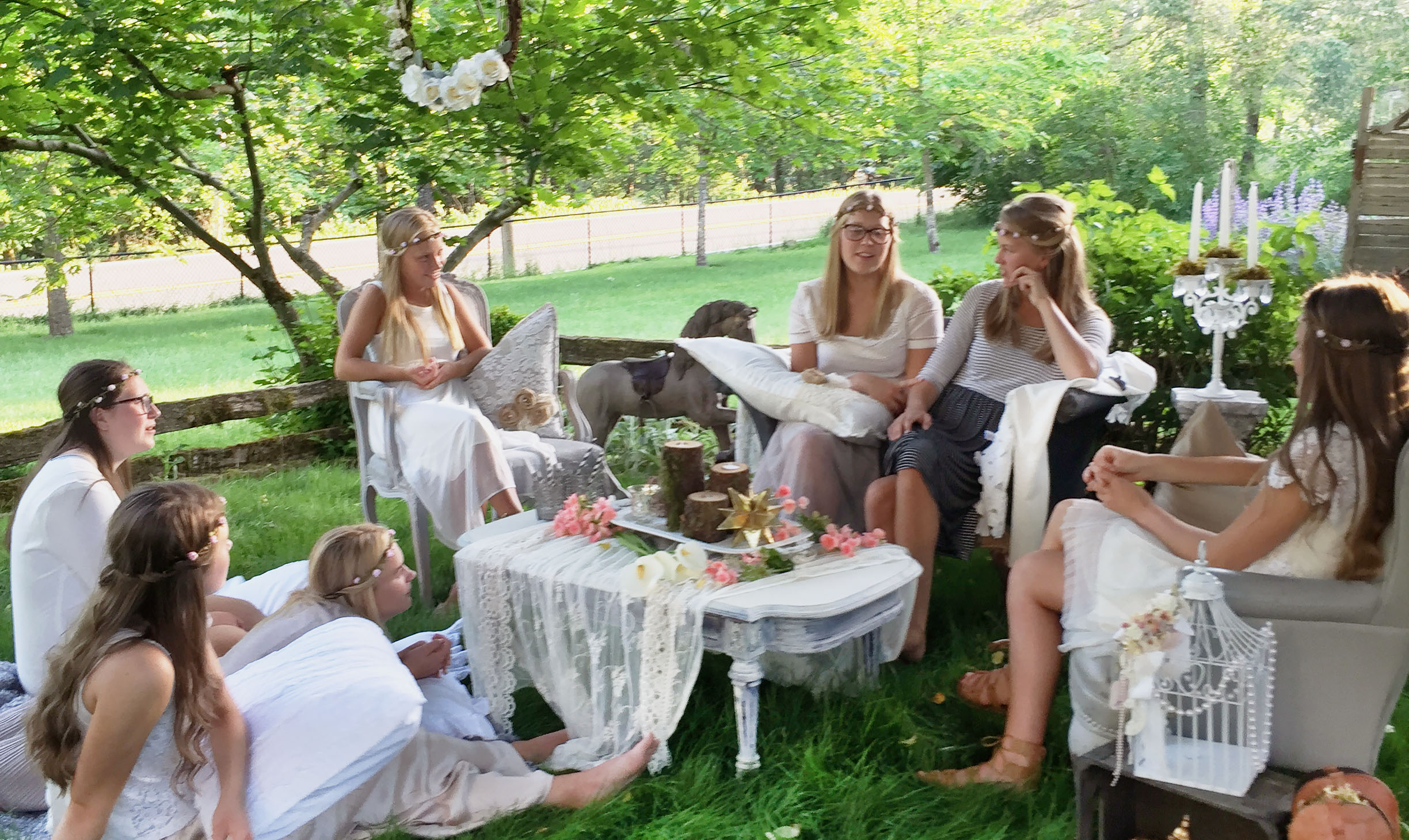This is a color photograph capturing an idyllic outdoor scene where a group of young women, likely either high school or college age, are seated around a short, white-painted wooden table. They are all dressed in flowing white dresses and adorned with floral crowns, suggesting a festive occasion such as a May Day celebration, sorority party, or bridal shower. The setting is lush with freshly mowed green grass and a backdrop of dense trees, through which sunlight softly filters from the top right. A white fence runs through the upper third of the image, adding a quaint touch. 

Central to the setting is a rectangular coffee table covered with a lace tablecloth. On the table sits a tray with candles and pink flowers, and possibly some beverages. Decorations, including white flowers, are placed above, enhancing the celebratory atmosphere. The seating arrangement includes two young women on a love seat, two in chairs placed at the head and end of the table, and three more on the ground—one lying down and two sitting upright—engaged in lively conversation. To the right, a candelabra with candles adds an elegant detail to the scene.